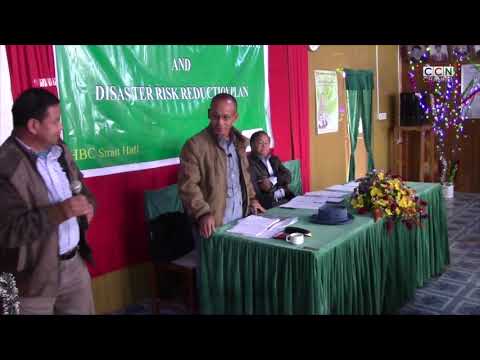This photograph captures a meeting or function featuring three African-American men, all dressed in formal attire. Central to the image is a man standing in a dark suit with a blue shirt and tie, seemingly addressing the attendees. He appears solemn, with his head slightly bowed towards a bouquet of flowers visible at the bottom edge of the photo. Flanking him on either side are two seated men, their heads bowed, suggesting they might be praying. Both seated men are partially cut off by the black borders at the top and bottom of the image. Behind them, a banner in green and white, partially obscured, reads "Proposed Concept Plan of...", "and Master Risk Reduction." The background includes a map and various pictures hanging on the wall.